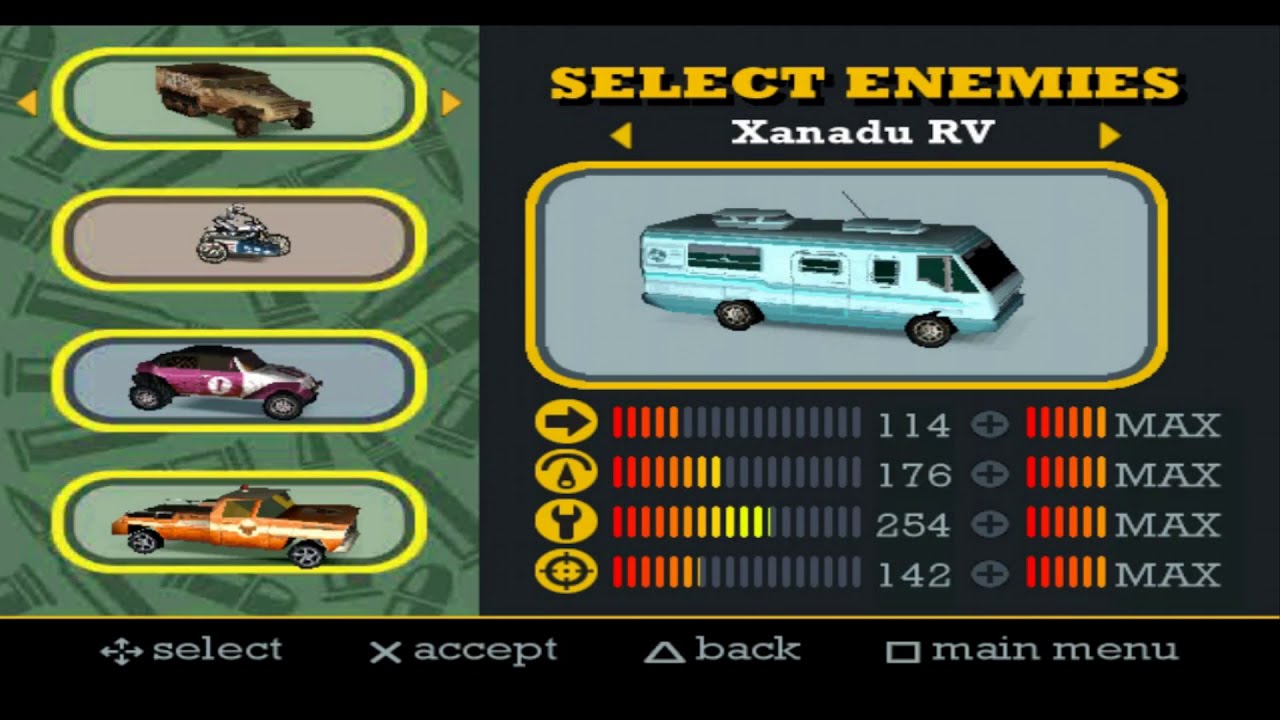The image depicts a screenshot from an auto-themed video game, where the player is in the vehicle selection screen. At the top of the screen, in golden letters, it says "Select Enemies." Directly below this, there are white letters spelling out "Xanadu RV," flanked by gold triangles pointing to the left and right. The selected vehicle, an old 70s RV, is displayed prominently in a central region bordered by a yellow rectangle with a gray background.

Below the vehicle image, the RV's performance stats are carefully detailed. There are various icons indicating different attributes: an arrow pointing to the right with a rating of 114 and red and orange bars, a wrench with a rating of 254 and red, yellow, and gray bars, and a bullseye icon rated at 142 with corresponding colored bars. Another metric, presumed to be fuel, is noted to have a value of 176.

On the left side of the screen, alternative vehicle options are lined up for selection, including a military Jeep, a motorbike, a four-wheeler with large tires suitable for off-road, a car, a purple and white monster truck, an orange pickup truck, and an army tank. At the very bottom of the screen, there is a black section housing the options to Select, Accept, Go Back, or return to the Main Menu.